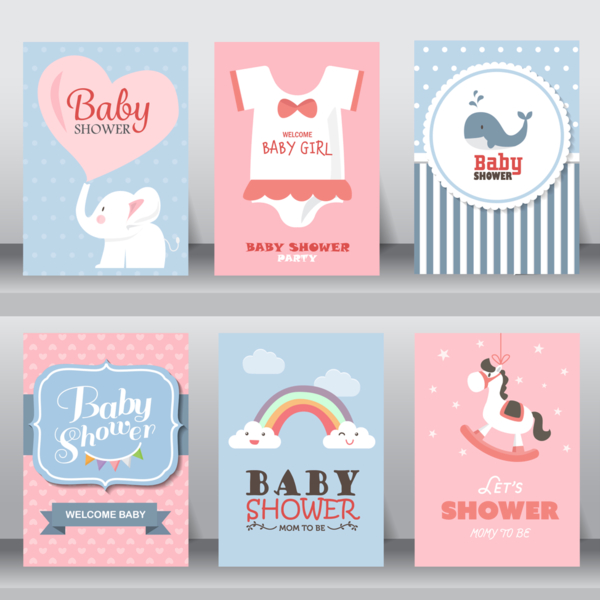The photo displays six baby shower invitations arranged in two rows of three on dark gray shelves against a light gray background. 

1. **Top Left**: A blue and white polka-dotted card featuring a white elephant with a pink heart from its trunk, inscribed with "Baby Shower" inside the heart.
2. **Top Center**: A pink background card displaying a white and pink ruffled onesie that reads "Welcome Baby Girl, Baby Shower Party."
3. **Top Right**: A card with a blue and white striped bottom and a blue and white polka-dotted top, featuring a blue whale in a round cut-out circle that says "Baby Shower."
4. **Bottom Left**: A pink background card adorned with white and pink hearts, a blue border stating "Baby Shower," and another smaller border that says "Welcome Baby."
5. **Bottom Center**: A blue background card with two clouds connected by a rainbow, labeled "Baby Shower, Mom to Be."
6. **Bottom Right**: A pink background card with white stars and a rocking horse ornament hanging from the top, reading "Let's Shower Mommy to Be."

The invitations reflect both gender-specific themes and neutral designs, showcasing a mix of blue and pink elements.